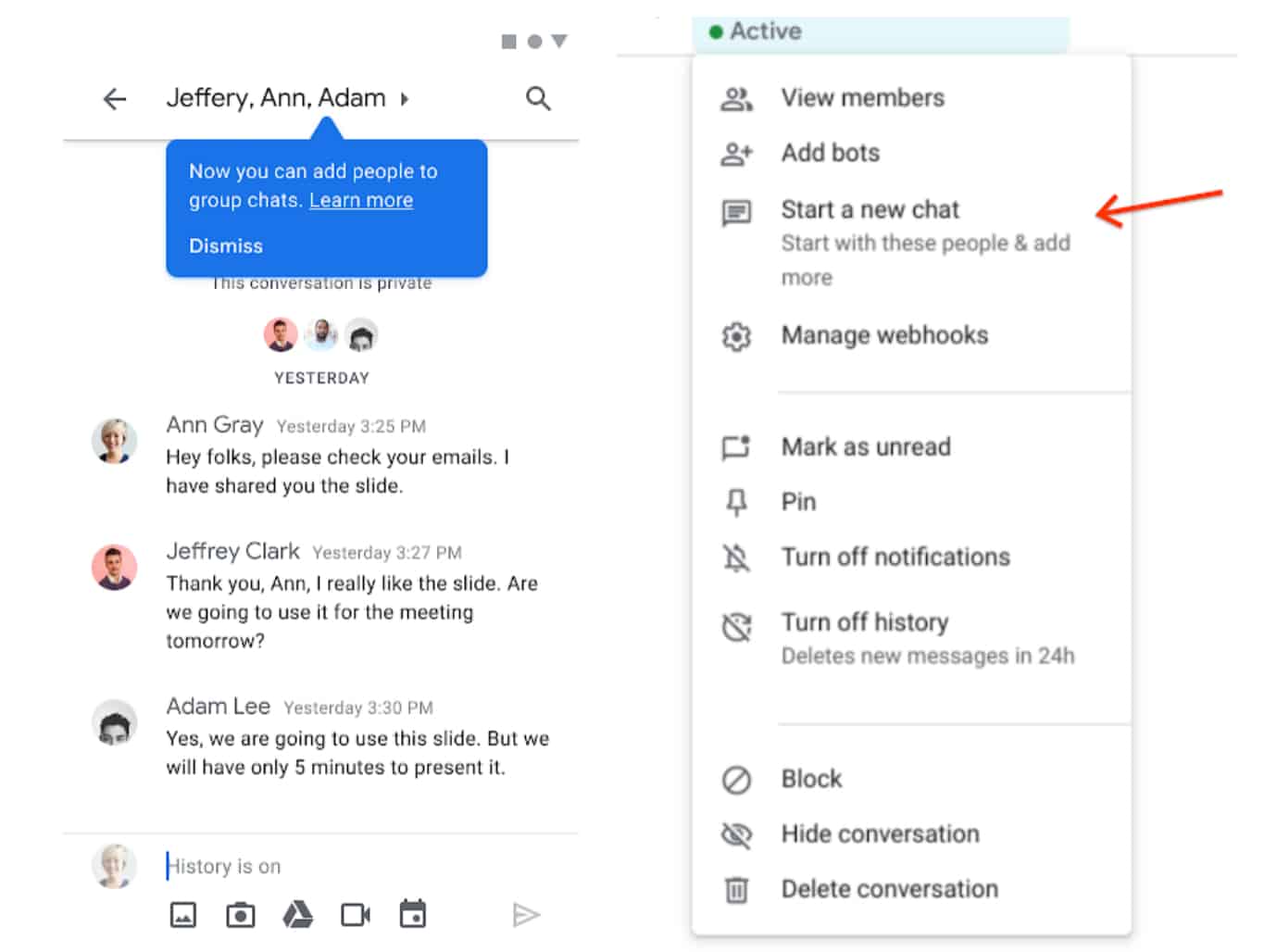This image is a screenshot of a collage featuring two distinct sections. On the left side, there is a chat interface with a white background. At the top of this section, there's a header with a left-pointing arrow, followed by the names "Jeffrey, Ann, Adam" written in sequence. Adjacent to these names, there is a gray right-pointing arrow, and further to the right, a gray magnifying glass icon.

From the first 'A' in "Adam," a blue speech bubble extends downward with white text reading, "Now you can add people to group chats. Learn more," the latter part underlined, and a "Dismiss" option situated to the right. Below this notification, the chat content starts with the phrase "This conversation is private."

Underneath, three profile pictures are displayed, followed by the timestamp "Yesterday." The chat log begins with a profile picture of a woman labeled "Ann Gray," accompanied by a timestamp of "Yesterday, 3:25 p.m." and a message reading, "Hey folks, please check your emails. I have shared the slide."

Next, a profile picture of a man is shown alongside the name "Jeffrey Clark," timestamped "Yesterday, 3:27 p.m." with the message, "Thank you, Ann. I really like this slide. Are you going to use it for the meeting tomorrow?"

Subsequently, a profile picture displaying the top of a man's head appears with the name "Adam Lee," timestamped "Yesterday, 3:30 p.m." and a message stating, "Yes, we're going to use this slide, but we only have five minutes to present it."

A thin gray line follows, beneath which there is a text entry box with the placeholder text "History is on." To the left of this box is the grayed-out profile picture of the initial chatter, accompanied by a blue cursor positioned at the beginning of the text box.

On the right side of the collage, there is a drop-down menu, but its details are not specified in the provided description.